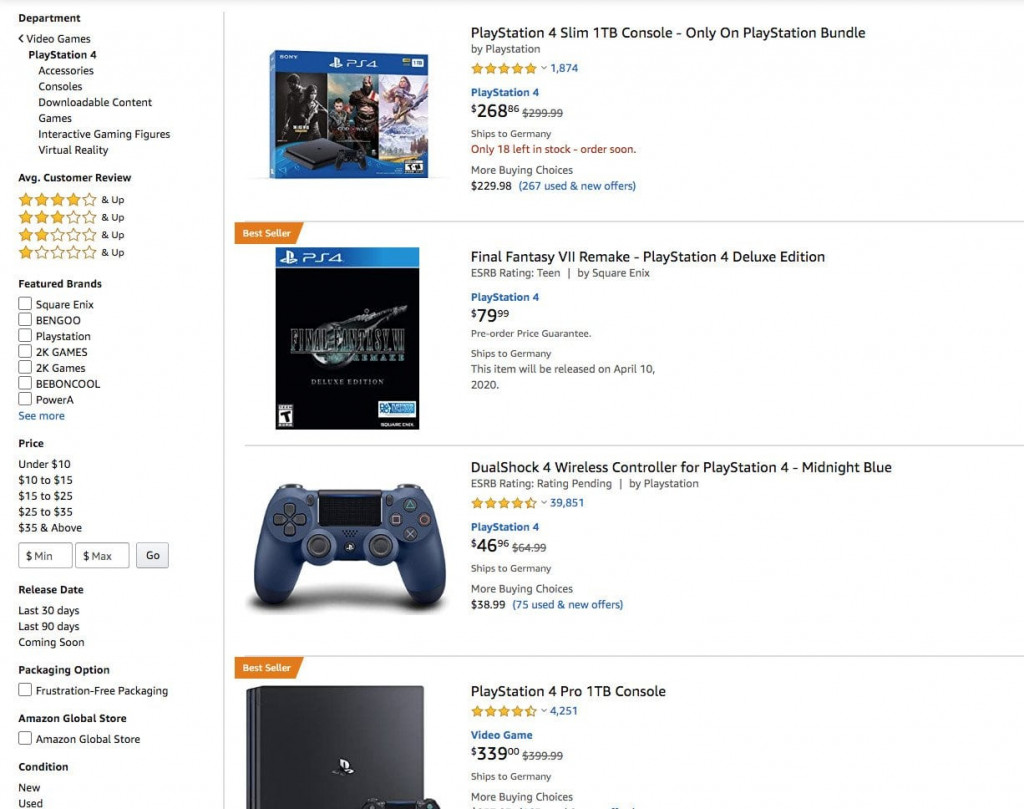The image displays an Amazon search results page for 'PlayStation 4' under the 'Video Games' department. On the left sidebar, categories are listed including 'Accessories,' 'Consoles,' 'Downloadable Content,' 'Games,' 'Interactive Gaming Figures,' and 'Virtual Reality.' Below this, there is a section for filtering by 'Average Customer Review,' followed by 'Featured Brands,' although the text appears small and difficult to read clearly.

The search results showcase several items, starting with the 'PlayStation 4 Slim 1TB Console - Only on PlayStation Bundle by PlayStation,' which has a 5-star rating based on 1,874 reviews and is priced at $268. Beneath it, there is the 'Final Fantasy VI Remake - PlayStation 4 Deluxe Edition.' Following that, the list includes the 'DualShock 4 Wireless Controller for PlayStation 4 - Midnight Blue.'